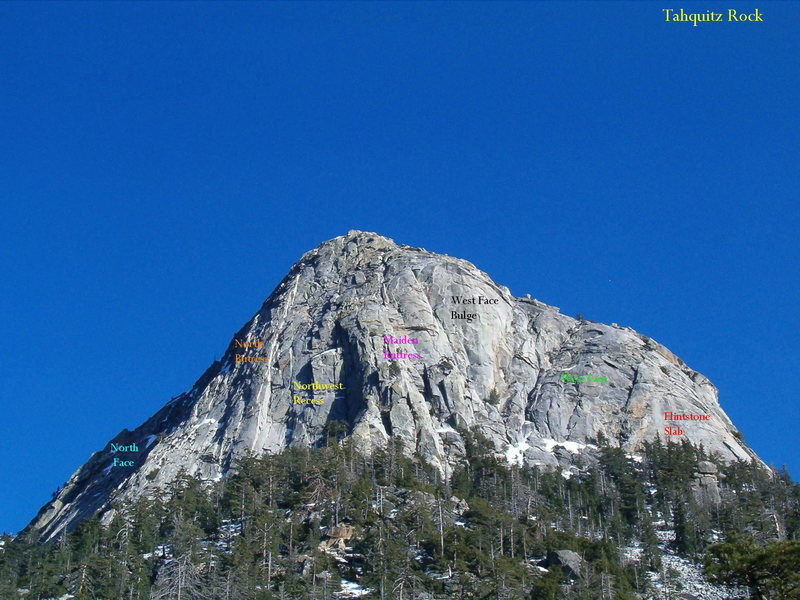The image is a detailed photograph of Tahquitz Rock, prominently labeled in the top right corner. The mountain features a rugged grey and stony appearance, accented by various colored labels indicating different sections of the formation. On the left side, "North Face in Shadow" is written in blue. The center-left showcases "Northwest Recess" in yellow. Moving towards the center, "Blintone Slab" is identified in red, while the upper right corner notes "West Face Bulge" in black. Additional labels are seen but are challenging to read, including an orange one towards the upper center and a green one on the middle right side. Below the mountain lies a dense growth of trees, and the backdrop reveals a vibrant blue sky, with the camera angled slightly upwards to capture the imposing rock formation and the immediate hillside. The image overall presents a clear, insightful depiction of the landscape.